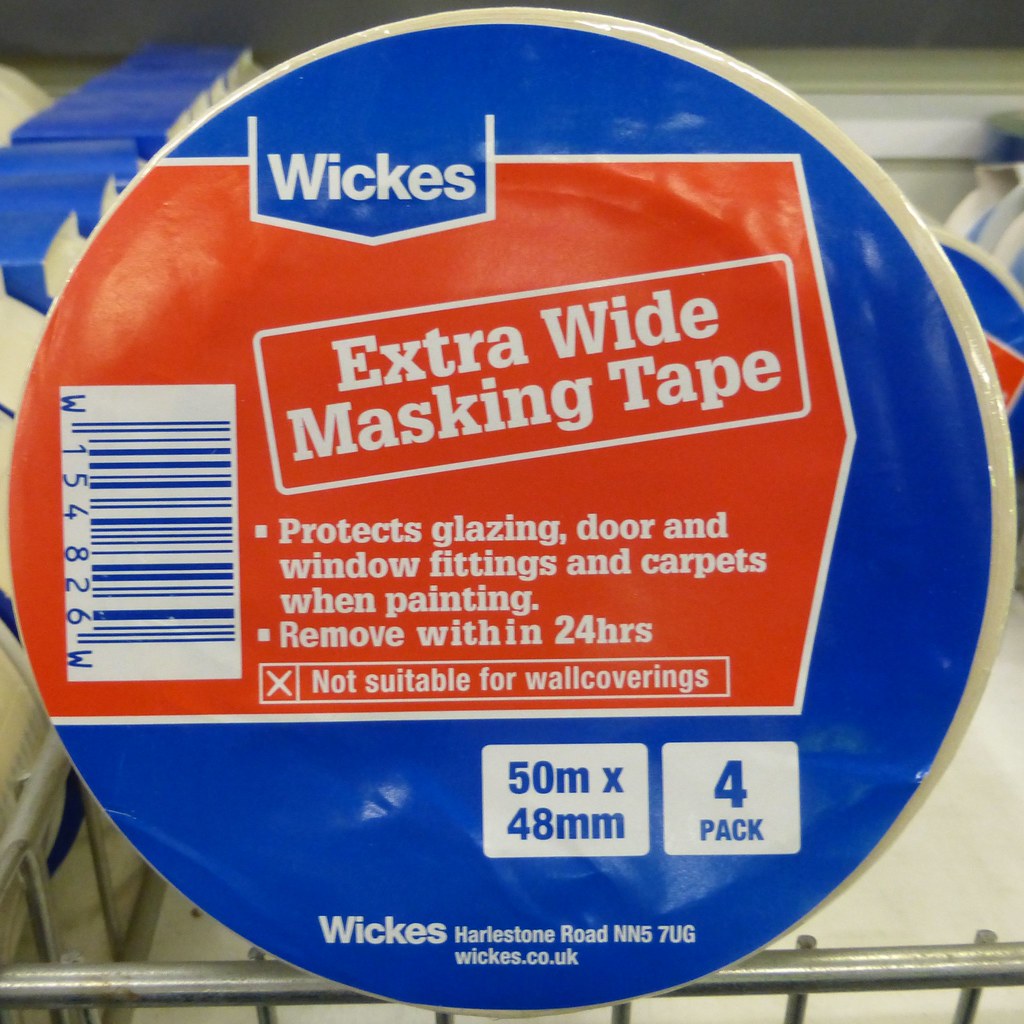This is a very detailed color photograph, formatted as a square, capturing a close-up shot of a roll of masking tape still in its packaging. The tape is in a store, as evidenced by the visible bottom portion of a shopping cart in the background. The roll itself is a round design, with a prominent label comprising red, white, and blue colors.

The label features a red rectangular panel prominently on the left side, with a white interior and white text that reads "Extra Wide Masking Tape." Above this panel, a blue arrow points downward with the brand name "Wix" in white text. Additional product details follow in white text: "Protects glazing, door and window fittings and carpets when painting. Remove within 24 hours. Not suitable for wall coverings."

Underneath the roll in the center, there are two bullet points listing benefits of the product. A blue background at the bottom of the label reads the dimensions "50 meters by 48 millimeters," and further down, it indicates the tape is part of a "4-pack." The very bottom of the label contains an address in white text: "Wix Harleston Road NN57UG Wix, Dakota, UK."

The style of the image can be described as Photographic Representationalism Realism, with a clear focus on depicting the product's packaging design.